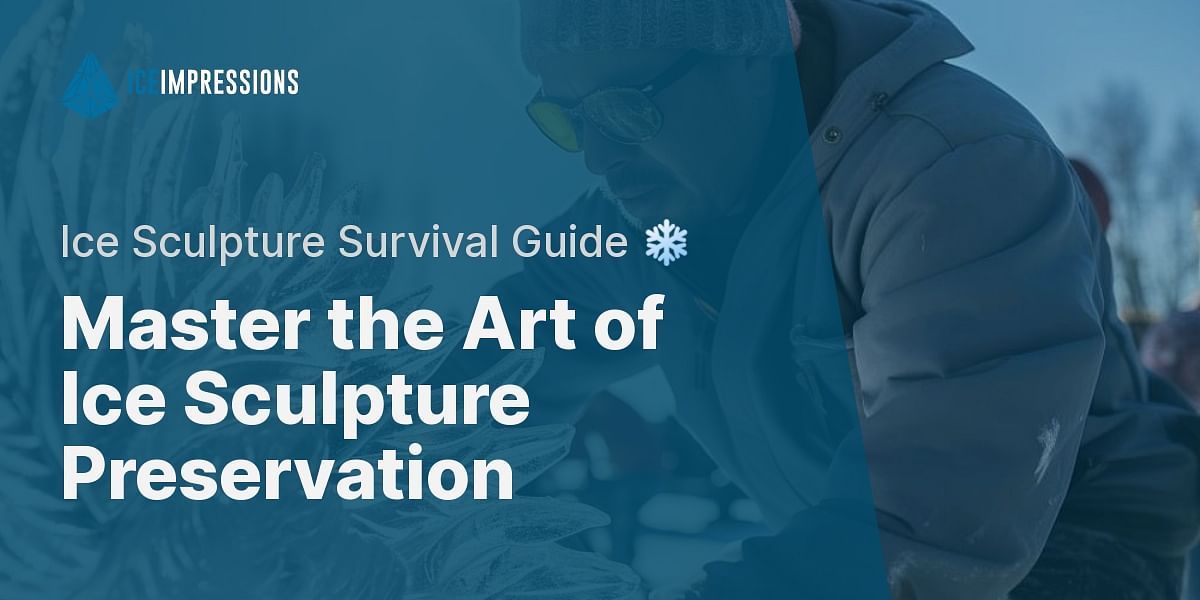This is a horizontal advertisement, possibly a poster or booklet cover, featuring a photograph with a green-blue filter overlay. The overlay, a slanted rectangle, partially obscures the background and contains text about ice sculpture preservation. At the top left corner, the logo "Ice Impressions" is displayed in small white capital letters next to a blue icon. Dominating the central part of the overlay, the white text reads "Ice Sculpture Survival Guide" accompanied by a grey snowflake icon. Below this, in bold white lettering, the phrase "Master the Art of Ice Sculpture Preservation" is prominently featured. The background shows a man clad in a grey winter coat, wearing safety glasses and a ski cap, possibly with a mustache, concentrating on an elaborate ice sculpture. The setting appears to be outdoors with trees and a building faintly visible behind him through the tinted overlay. The overall color theme is predominantly blue, giving the entire advert a cool, frosty ambiance.